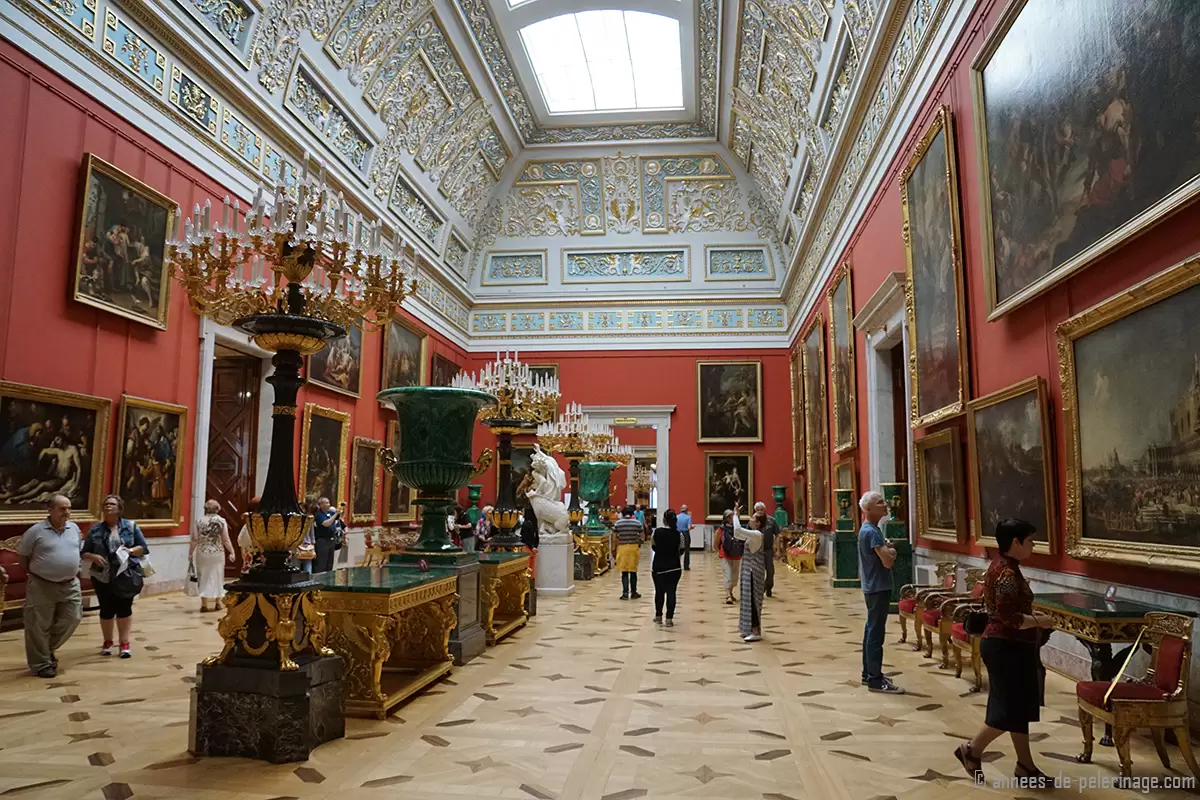The image depicts the interior of an elaborately decorated, European museum, possibly reminiscent of the Louvre. The room is a large, ornate foyer with a ceiling adorned with intricate floral carvings and tiny silhouettes of men's faces, all painted in light blue with gold leaf embellishments. The ceiling features a large skylight that allows natural light to flood the space, highlighting the elegance of the architecture with its curves and detailed work. Below, the reddish-pink (or salmon-colored) walls showcase numerous Renaissance-era paintings, primarily of religious scenes, each framed in gold. The museum room also has antique-style chandeliers with crystal and candle-like lights hanging from black poles. Several period tables and decorative chairs are arranged around the room, including a prominent table in the center displaying a large green urn, possibly made of jade. The space is paved with wooden floors in diagonal patterns, and there are several visitors in summer attire, milling about, observing the art and taking photographs.